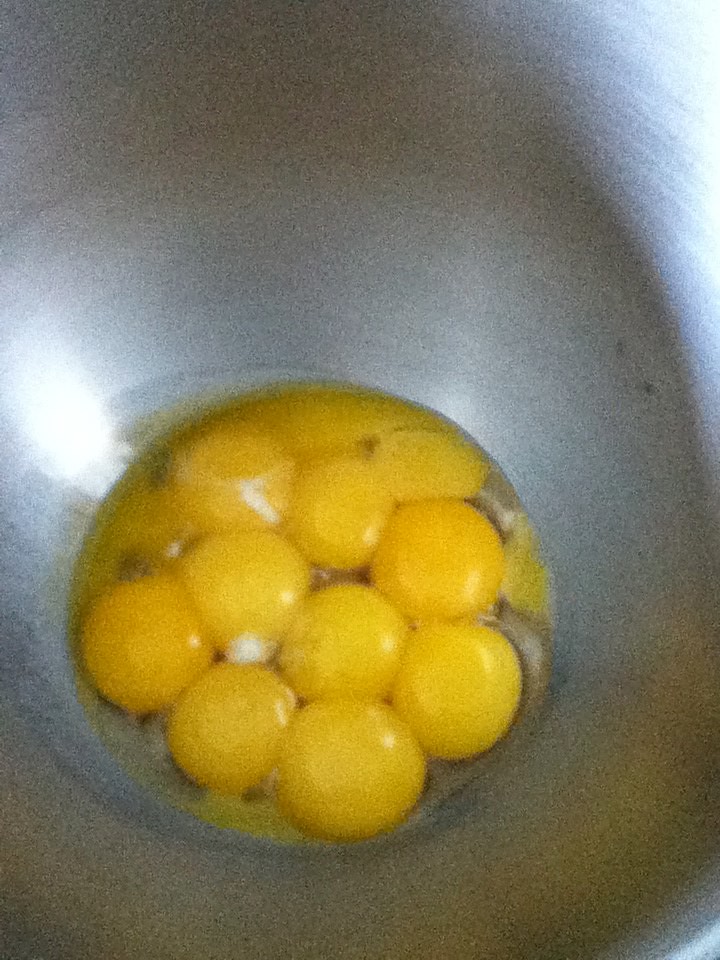This close-up photograph captures the inside of a silver metal bowl. The entire picture focuses on this bowl, which has a narrow, deep bottom. At the bottom, there are approximately 9 to 11 raw egg yolks, all mostly intact, though one appears broken. The yolks are vivid yellow and arranged in a circular formation. There's a faint presence of egg white around a few of the yolks, but the focus is primarily on the rich yolks gathered at the bottom. The shine of the metal bowl and the bright yellow of the yolks dominate the image.